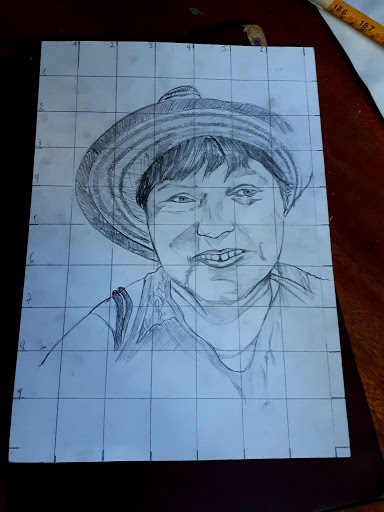The image is a photograph of a pencil sketch, slightly taller than it is wide, resting on a dark brown table with a black cloth on it. The sketch is done on a piece of white paper with large grid lines, approximately seven squares across and ten squares down, for easier drawing precision. In the top right corner of the scene, there is a white piece of paper and a pencil lying across it. The subject of the drawing is a friendly-looking man with medium-length dark hair and a wide smile revealing crooked teeth. He dons a straw hat with decorative lines and a casual shirt featuring an open-necked collar. The man’s eyes are open, giving a warm, approachable expression. Some parts of the sketch display gray toning techniques, and the overall piece appears somewhat grubby, indicating that charcoal may have been used as well.